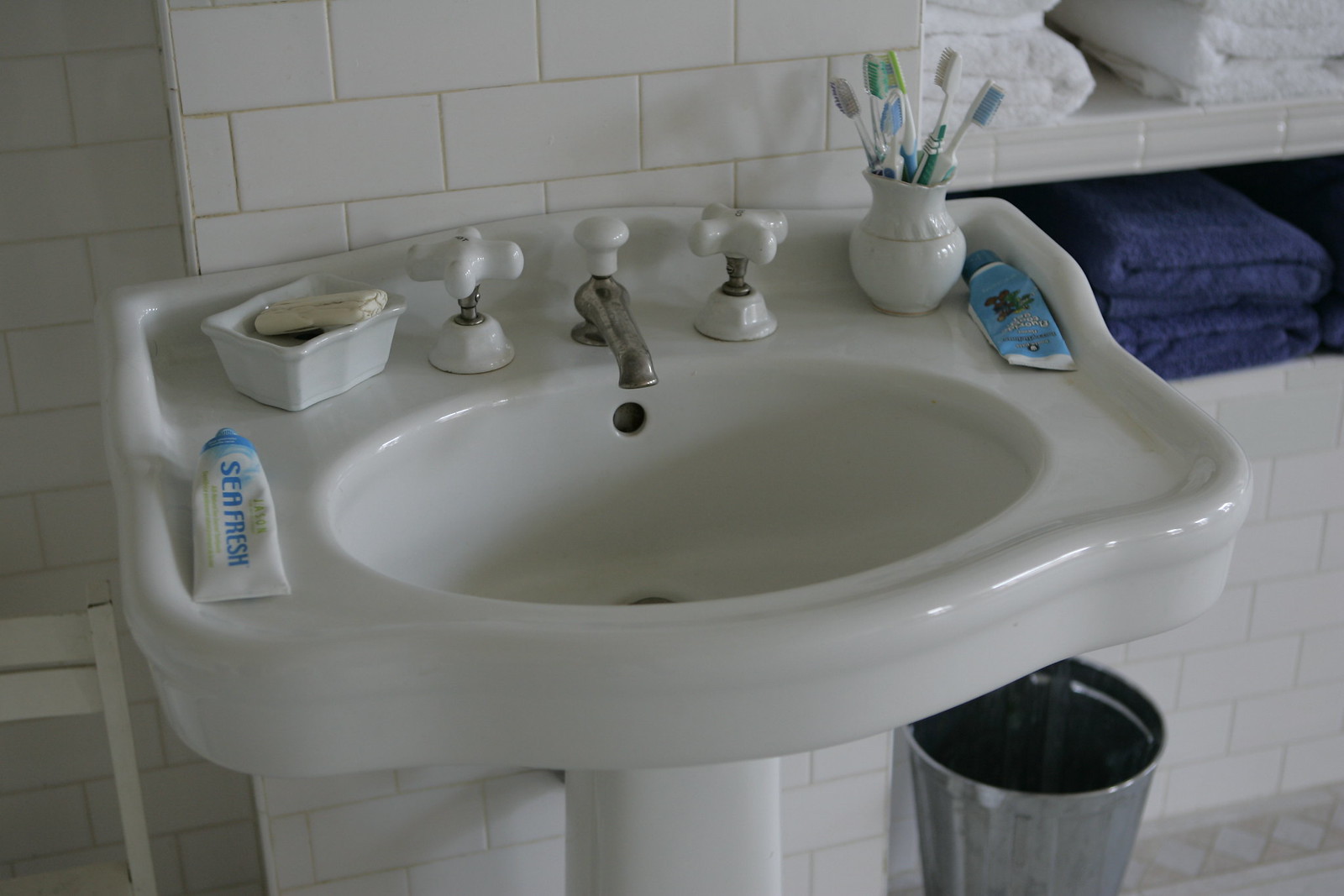This color photograph captures a close-up view of a bathroom sink area. The surrounding walls, adorned with light gray tiles, provide a clean and modern backdrop. In the upper right corner, a shelf adds both functionality and aesthetic. The top shelf neatly holds a couple of pristine white towels, while the shelf below features two slate blue towels, carefully folded.

The sink, made of porcelain white, is complemented by a chrome faucet. The hot and cold water handles, matching the sink in porcelain white, enhance the cohesive look. Sitting atop the sink is a large, white vase serving as an unconventional toothbrush holder, housing six manual toothbrushes.

To the right of the vase, a turquoise blue tube, likely containing toothpaste, stands visible. On the left side, we find a distinctly identified tube of Aquafresh toothpaste, characterized by its white tube and turquoise blue lettering. A small white soap dish holds a matching white bar of soap, completing the neatly organized sink area.